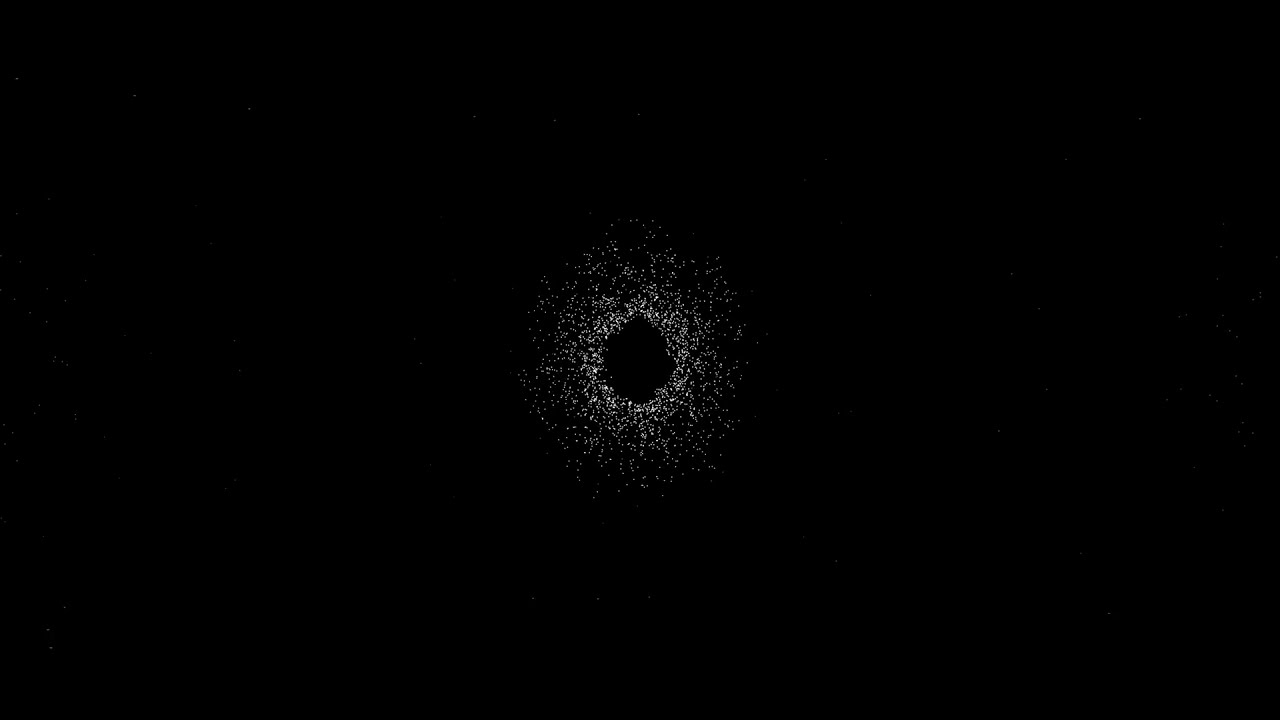The image is predominantly black and rectangular, with a notably detailed center. At the heart of the image lies a black hole, centrally located, serving as the focal point. Surrounding this black void is a dense concentration of white dots, almost forming a donut-like shape with the black hole as the hole in the middle. These pinpoints of light are densely packed immediately around the black hole and gradually thin out as they spread further away. The black hole itself appears with slightly varying descriptions, resembling shapes such as a Hershey kiss, a Christmas tree, or a bell. Amidst the surrounding expanse of black, a sparse scattering of faint white specks can be observed, becoming more dispersed farther from the center, creating an impression of a radiant core gradually fading into the dark void.